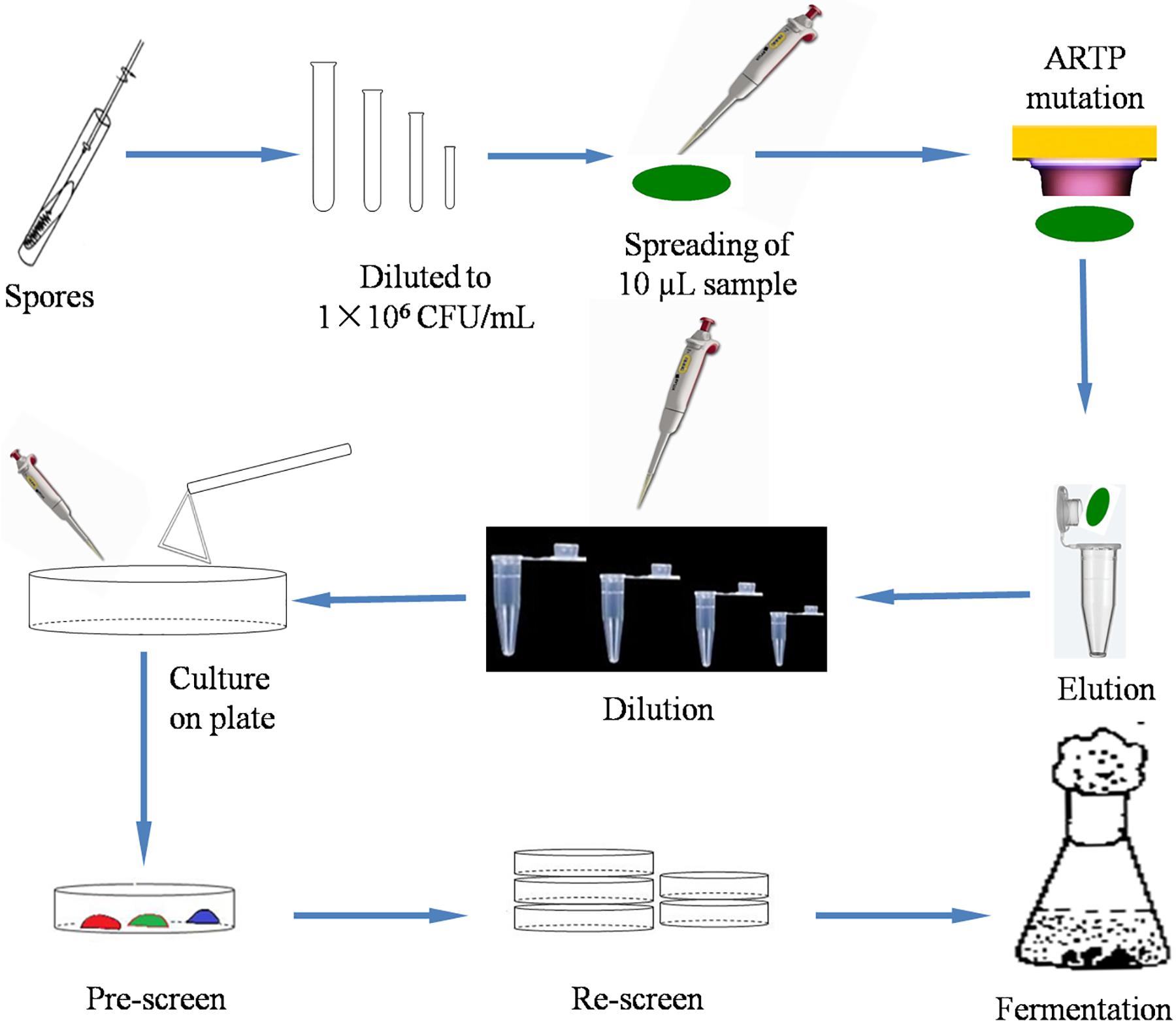The scientific diagram illustrates a detailed experimental procedure for manipulating spores through various stages. It starts at the upper left with an image of a vial containing spores, labeled "spores." A blue arrow guides to the next step, showing four progressively smaller test tubes beneath the label "diluted to 1x10^6 CFU/mL." The process continues with an arrow pointing to a green oval representing sample spreading, followed by another to the "ARTP mutation" stage depicted with a yellow rectangle on a pink cylinder.

Next, a blue arrow leads to a step labeled "elution," illustrated by an open vial receiving a green oval. The process continues downward with an arrow pointing to "dilution" and a series of five Petri dishes—three stacked and two separate. Another step, "culture on plate," leads to the observation stages: "prescreen," showcased with a Petri dish containing red, green, and blue semi-circles, and "rescreen." Finally, the last arrow points to "fermentation," depicted by a beaker with black dots, symbolizing the end of the experimental sequence.